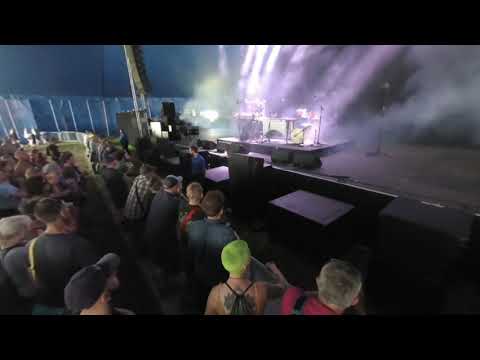The image captures a moment just before the start of a musical performance, likely taking place indoors under a blue tent awning. The stage, located on the right side, is enveloped in a haze of fog or smoke that glows with purplish and bluish hues, obscuring the performers from view. Musical equipment is clearly set up on a black platform. Overhead lights cast their rays on the stage, enhancing the scene's atmospherics. The audience, positioned on the left, consists mostly of seated individuals, all intently watching the stage in anticipation. Among the crowd, a few stand-out features include a person with dyed light green hair, a man in a red shirt with a strap over his left shoulder, and another wearing a black cap in the foreground. The background reveals structural details like support poles and possibly a fence. Main color tones in the image are dominated by black, white, with accents of light green, pink, and blue. The top and bottom of the image are bordered by black bars, focusing attention on the central scene.